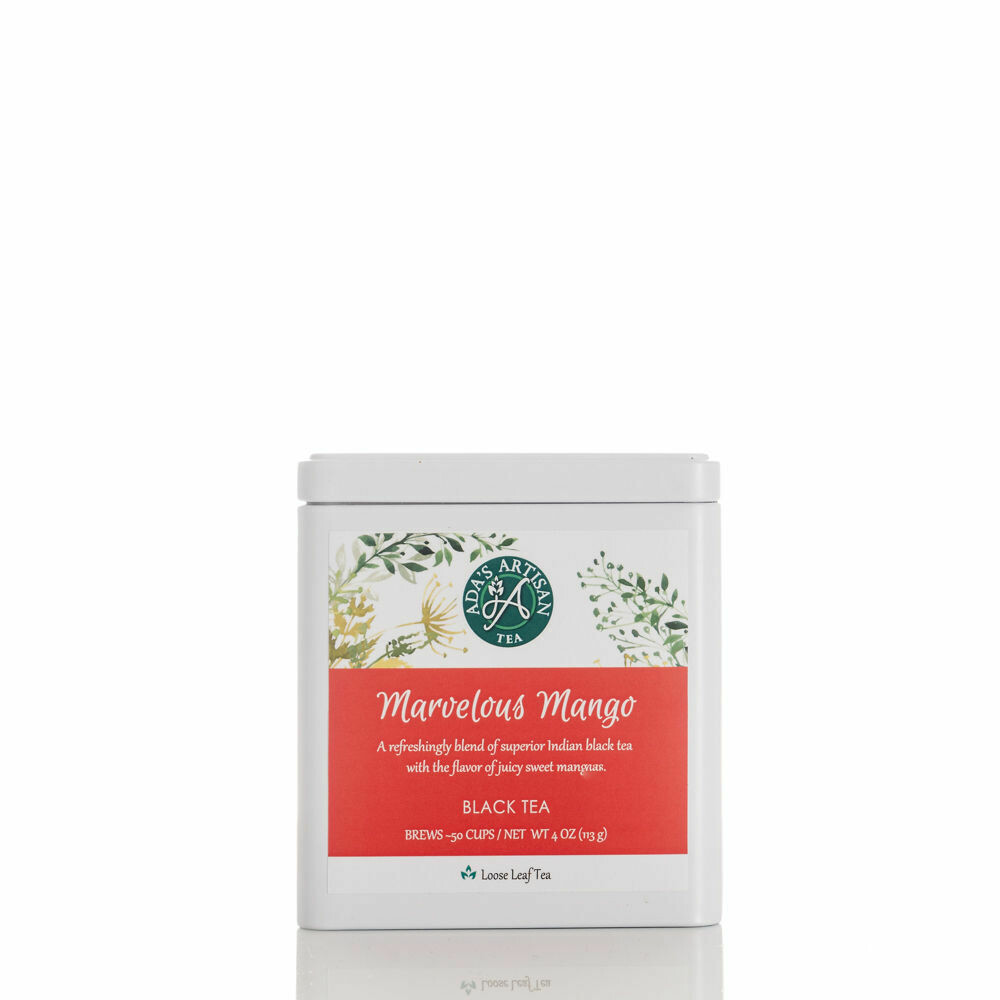This close-up photograph features an attractive white tea tin with a botanical-themed design, displaying illustrations of leaves in various shades of green and yellow. The tin is primarily white, with a notable label. The label is divided into two sections: the top half is white and the bottom half is a dark orange. At the top center of the label, within a green circle, the text "Ada's Artisan Tea" is printed in white letters with a cursive "A" and botanical motifs flanking it. Below, on the orange background, the name "Marvelous Mango" is prominently featured in white fancy script, alongside a description that reads: "A refreshing blend of superior Indian black tea with the flavor of juicy sweet mangoes." Beneath this, in all caps, it states "Black Tea," and further down, "Loose Leaf Tea" is noted in black letters. The background of the image is completely white, drawing full attention to the elegant design of the tea tin.